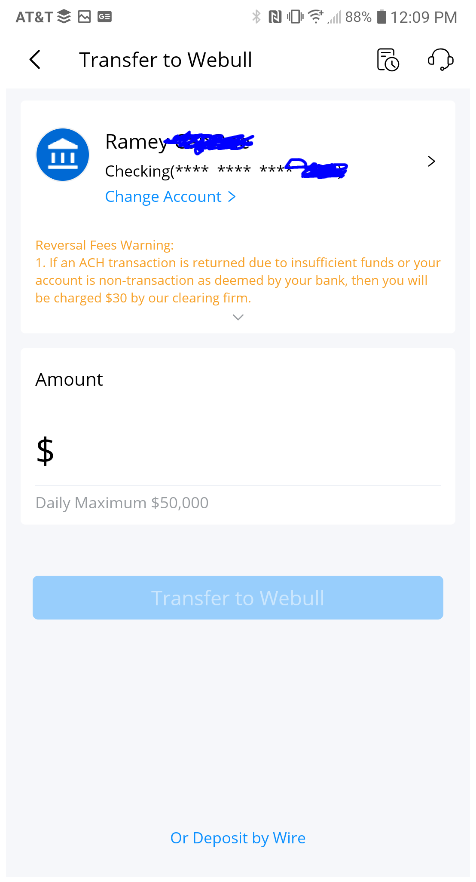**A screenshot taken from a mobile phone's interface shows a transaction screen for transferring funds to a Webull account. At the top of the image, "Transfer to Webull" is prominently displayed. Under this header, the text "Ramey" is visible, with the rest of the name obscured with blue marker for privacy. Below this, the account details are partially censored with asterisks and more blue scribbles, concealing all but the last four digits of the account number. The section labeled "Checking" is similarly redacted. 

As the screen continues down, the option to "Change Account" is available. Following this, a warning about reversal fees indicates that a $30 charge may apply if an ACH transaction fails due to insufficient funds or a non-transactional account. The following section, labeled "Amount," is presented in black print, with a note that the daily maximum transfer limit is $50,000. 

A prominent button labeled "Transfer to Webull" sits near the bottom of the screen. Beneath this button, there is a gray, empty space preceding the final option, "Or deposit by wire," which is displayed in blue text. This detailed configuration of the interface ensures the user is aware of the transaction steps and related conditions.**